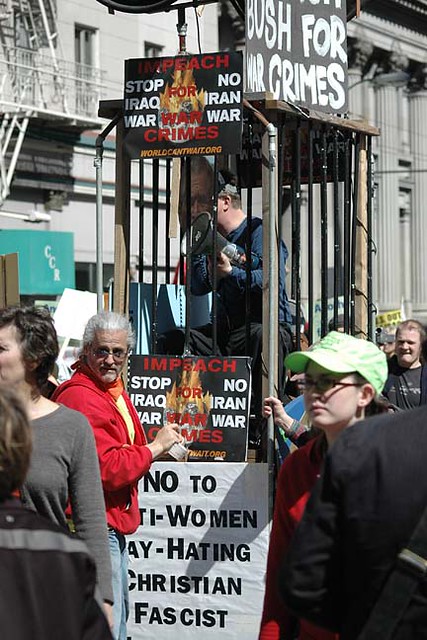In this vibrant outdoor daytime rally, a diverse crowd is gathered, clearly visible at the bottom of the image. They are holding up numerous protest signs with impassioned messages such as "Impeach for War Crimes," "Stop Iraq War, No Iran War," and "No to Anti-Women, Gay-Hating, Christian, Fascist." Prominent signs include "Bush for War Crimes," positioned above a central wooden cage structure that houses a man with a megaphone, clad in a blue top and black pants, drawing the eye directly to the middle of the image.

The crowd includes notable figures: on the bottom left, there's a person with their back to us, standing next to someone facing left, partially obstructed, whose head turns back towards the camera, revealing glasses and gray hair. Nearby, a woman in a red top and greenish cap faces forward, her glasses catching the light, while just to her right, a shoulder and arm clad in black enter the frame. Behind this lively scene, various buildings form the backdrop, featuring distinctive elements such as a fire escape to the left and vertical pillars to the right. The rally's vivid color palette includes shades of red, orange, green, blue, white, black, and gray, adding to the dynamic atmosphere of this detailed protest scene.